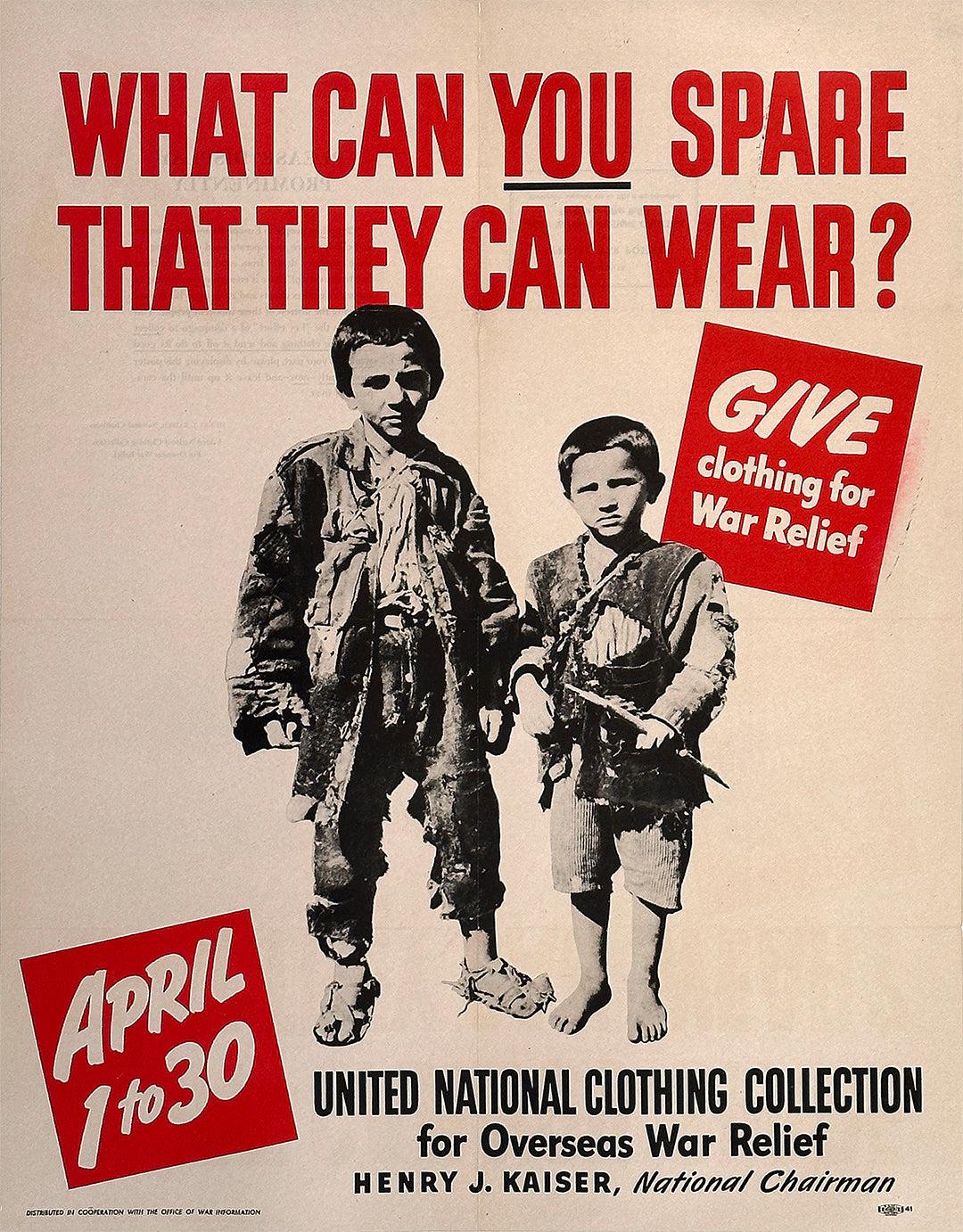This poster for the Relief Foundation features a striking image of two little boys with short hair, captured in black and white. The taller boy on the left is wearing makeshift sandals fashioned from a ripped-up shirt, while the younger boy on the right is barefoot. Both children are clad in heavily worn and torn clothing, highlighting their dire need for aid. 

The poster, which is vertically aligned and set against a light tan background, bears a powerful message at the top in large red, all-caps letters: "WHAT CAN YOU SPARE THAT THEY CAN WEAR?" with the word "YOU" underlined in black. To the right of the boys, a red box with white text urges, "GIVE CLOTHING FOR WAR RELIEF," emphasizing the immediacy of the need. 

On the lower left side of the poster, another red box with white text reads "APRIL 1 TO 30," indicating the timeframe for the clothing drive. At the bottom, in bold black all-caps, it states "UNITED NATIONAL CLOTHING COLLECTION," followed by "FOR OVERSEAS WAR RELIEF." The name, "HENRY J. KAISER, NATIONAL CHAIRMAN," is prominently displayed, lending authority and urgency to the campaign.

Overall, the poster visually and textually underscores the critical need for clothing donations to support children affected by war, encapsulating the essence of the Relief Foundation's mission.